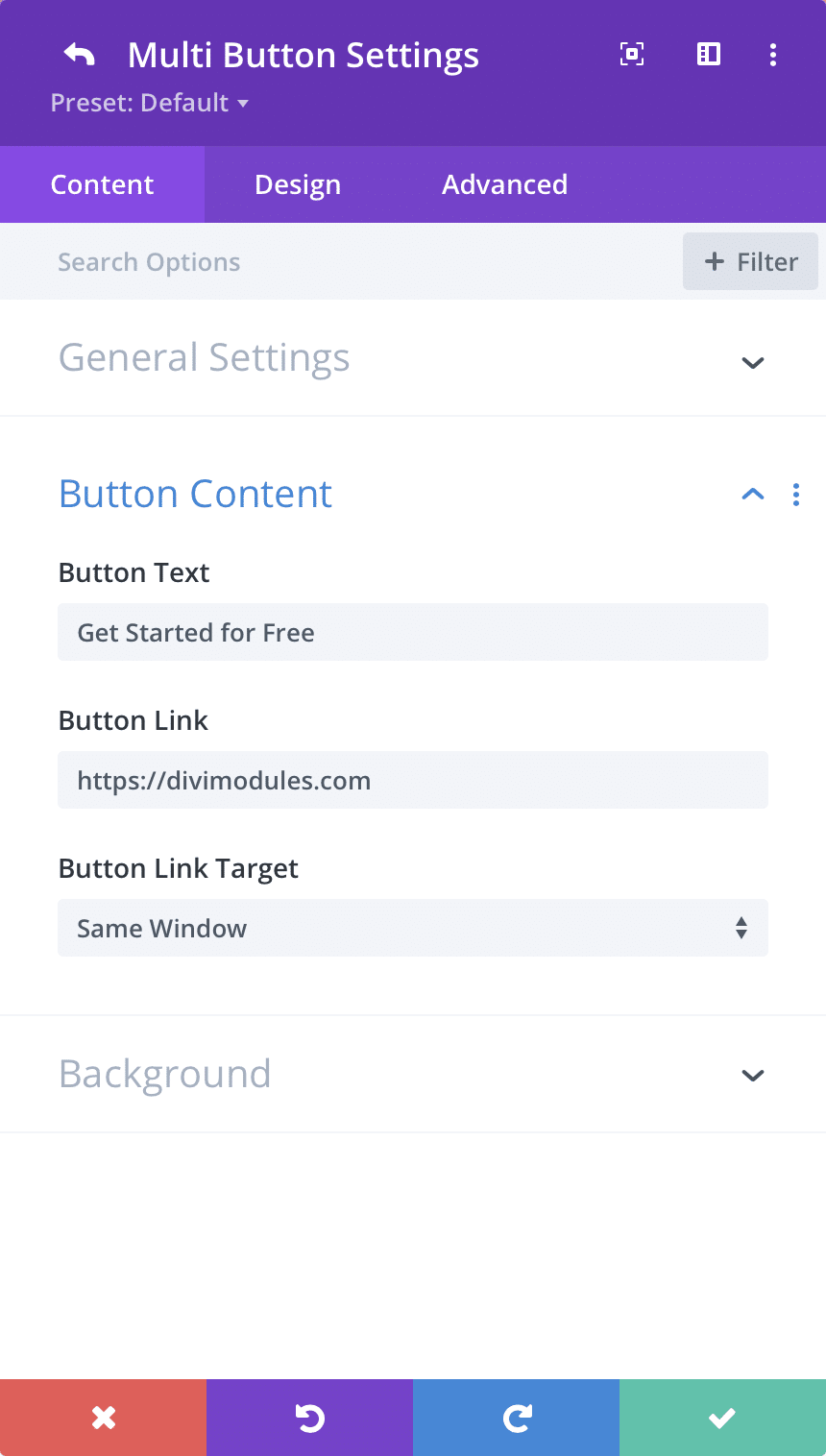The image displays a section of a website titled "Multi-Button Settings." The header of the website is a thick purple banner. Within this banner, the title "Multi-Button Settings" is prominently shown. Below the title, there is a "Preset Default" option accompanied by a white arrow that loops upward and to the left. 

At the top of the interface, just beneath the purple header, there are three tabs labeled "Content," "Design," and "Advanced." The "Content" tab is highlighted in light purple, while the other two tabs are the same shade of purple as the background.

Below these tabs, a gray search bar with the text "Search Options" is visible, featuring a "Plus Filter" option on the right side. Further down, the section labeled "General Settings" has a downward-pointing arrow next to it. Under this section, there is a "Button Content" option in blue. This section contains a text field labeled "Button Text" with the text "Get Started for Free" inside a box. There is also a "Button Link" field, which contains a URL, and a "Button Link Target" option set to "Same Window."

Continuing further down, there is a lightly printed "Background" section with a downward arrow next to it. The information then skips a bit, leading to the bottom of the website where four colored boxes are displayed.

These boxes include:
- A red box featuring an X.
- A purple box with an arrow circling around to the left.
- A blue box with an arrow circling around to the right.
- A green box with a checkmark.